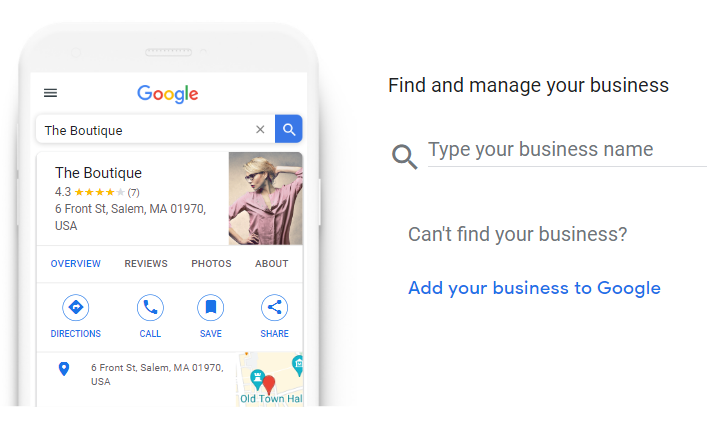This image is a detailed screenshot from a website featuring two distinct sections. 

On the right side, it showcases a clean, minimalistic interface with a white background, prominently displaying the text "Find and manage your business." Below this, there is a search field accompanied by a magnifying glass icon, with placeholder text prompting users to "type your business name." Just beneath this area, a supportive prompt reads "Can't find your business?" followed by a blue, likely clickable link stating "Add your business to Google."

The left side of the screenshot features a computer-generated image of a generic white cell phone. The phone screen displays a Google search interface. At the top, it shows the Google logo with a dropdown menu icon on the left. Below, the search field contains the typed query "the boutique," with a blue search button positioned to the right. The search results are visible underneath, starting with a listing for "the boutique," which is rated at 4.3 stars from seven reviews and includes an address. To the right of this listing, there is a photograph of a woman in a pink shirt posing like a model. Under this main listing, additional Google search results sections are visible, including "Overview," "Reviews," "Photos," and "About," along with several action icons for directions, calling, saving, sharing, and a link to Google Maps.